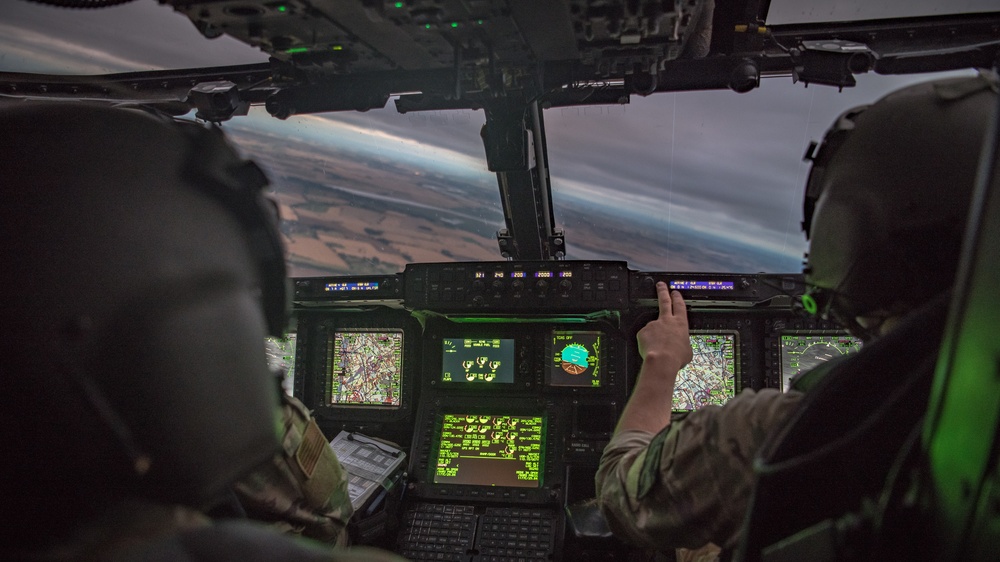The image captures a detailed view of the cockpit of what appears to be a military helicopter, potentially from a video game, based on the somewhat animated appearance of the occupants. Both the pilot and co-pilot, dressed in camouflage military uniforms with rolled-up sleeves and helmets, are seated with their faces unseen as they direct their attention out the windshield. The pilot on the right extends his left arm, with his fingers forming a peace-like gesture, possibly interacting with the controls. The cockpit is filled with an array of digital displays and control panels; one prominent screen in the lower center features bright green text, while other screens are adorned with various symbols and colors including tan, green, and red. The view out of the cockpit suggests the aircraft is tilting, revealing a landscape dominated by brown hues with patches of green and overshadowed by dark, dense clouds, indicative of a desert or sparsely populated area.